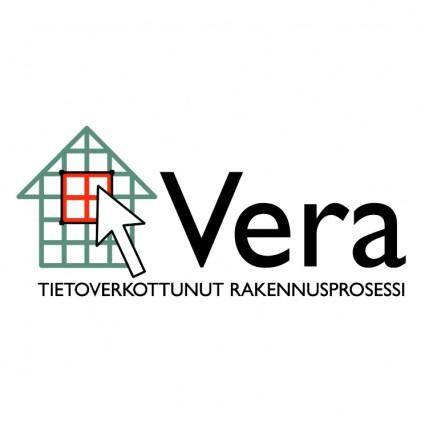The logo for the business is a detailed combination of typography and graphic design, arranged in a landscape orientation. On the left side of the logo, there is a graphical representation of a house outlined in green line squares, resembling a grid. The house features four central white squares outlined in red, representing windows, and is surmounted by an arrow shape pointing upward from the roof. Adjacent to the house, a large white cursor arrow points directly at the red-outlined window section. To the right of the house graphic, the company name "VERA" is displayed prominently in bold black letters. Below "VERA", there is a line of foreign language text in small black capital letters, possibly Cambodian, extending from the width of the house graphic to the end of the word "VERA". The logo's style integrates clean typography with illustrative elements, showcasing a harmonious blend of both.